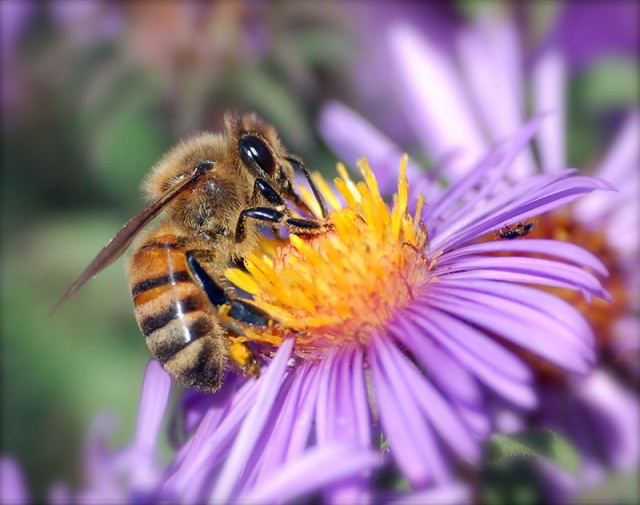This close-up photograph captures a honeybee diligently collecting nectar from the vibrant heart of a purple flower. The honeybee, positioned slightly left of center, is depicted with intricate detail, showcasing its characteristic black and orange striped abdomen adorned with light gray fur. The bee’s body features a striking black-tipped end, and its thorax bends subtly back to the right. The bee's wings, partly visible, sweep downwards towards the right. 

Engrossed in its task, the honeybee has its face buried deep within the flower's yellow interior, appearing to probe for nectar with its front limbs. The flower's structure is equally striking—lavender petals radiate from the vibrant yellow center, extending in various directions and becoming increasingly unfocused towards the edges. The flower's intricate stamen, adorned with fine white and yellow hairs, presents an appealing target for the bee. 

The background of the image provides a complementary blur of color, adding depth without detracting from the main subject. To the right, another purple flower peeks into the frame, out of focus but hinting at the surrounding floral environment. To the left, patches of green, ranging from light to dark, suggest a lush, verdant backdrop. Notably, a small bug clings to the underside of one of the purple petals, adding an intriguing detail to the scene's rich tapestry.